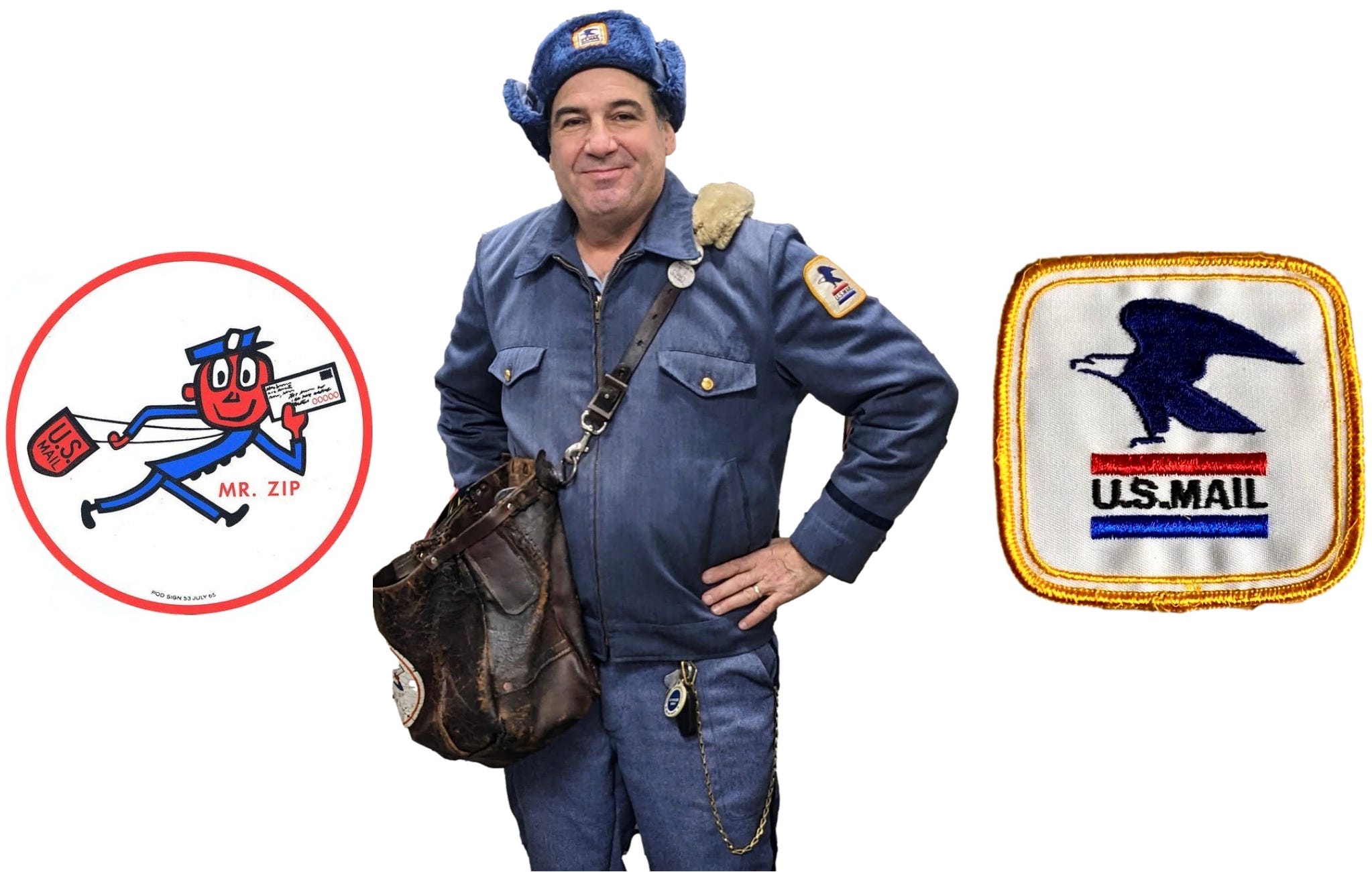The image depicts a vintage postal worker dressed in a classic uniform reminiscent of mid-20th-century mail carriers. The uniform consists of blue denim-like pants and a matching long-sleeved shirt that zips up the front and features two front pockets. A distinctive yellow patch adorns the shirt's shoulder. The detailed patch, shown separately to the right of the individual, features a gold border, a white background with red and blue stripes, the text "US Mail," and a bald eagle emblem colored in blue.

The postal worker carries a brown leather mailbag slung across his shoulder, resting against his hip. The bag prominently displays a logo of "Mr. Zip," a whimsical red character depicted in motion, holding a piece of mail and wearing a fuzzy blue hat while a U.S. mailbag trails behind him. The overall aesthetic captures the nostalgic essence of the postal service's bygone era.